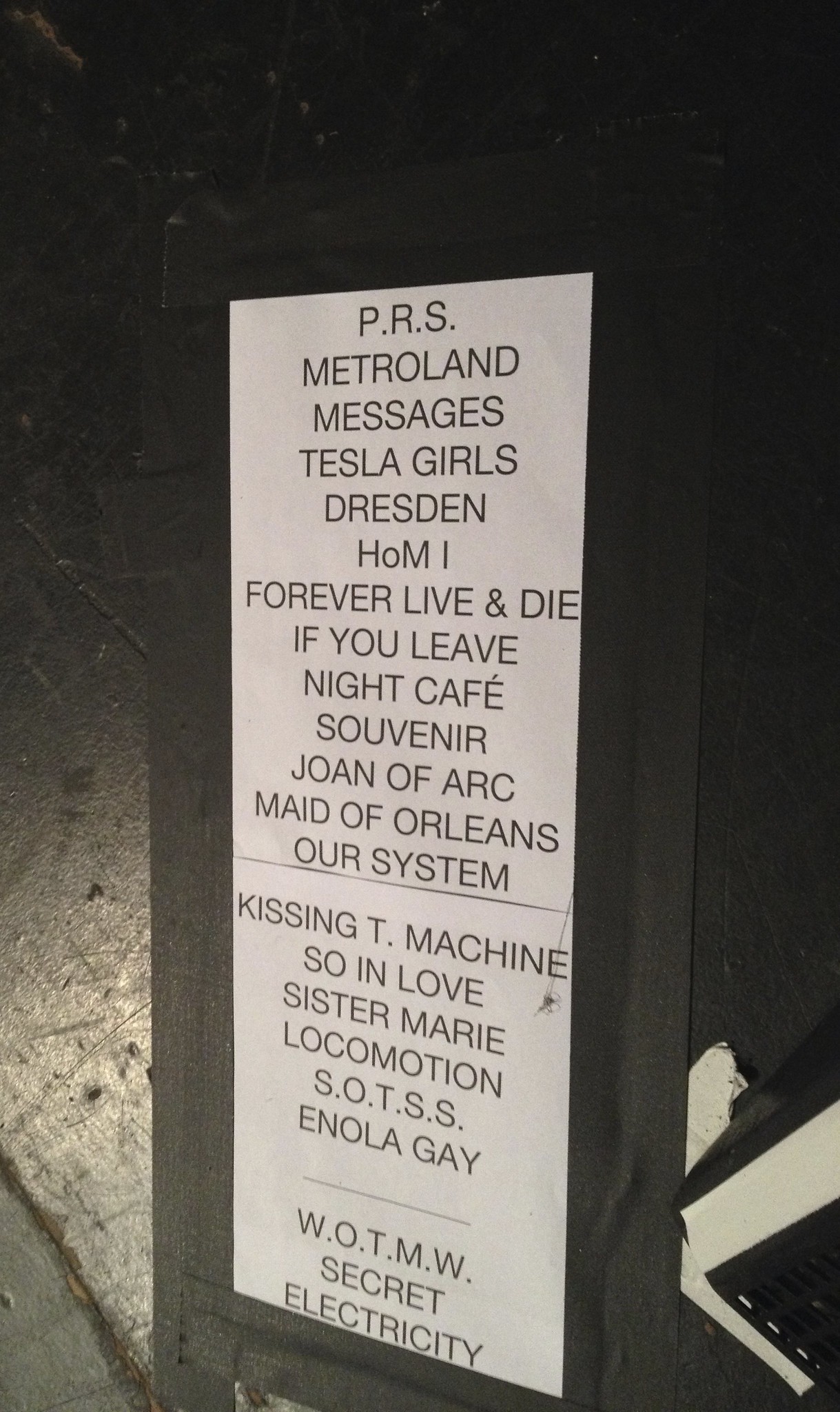The image features a tall, rectangular sign taped against a black, cement-painted wall with a shiny lower-left corner. The wall also has a white painted portion at the bottom right. The sign, printed on white paper, is bordered by thick, textured black tape and lists what seems to be names of musical acts or song titles in all capital black letters. The list, from top to bottom, includes: PRS, Metroland, Messages, Tesla Girls, Dresden, H-O-M-I, Forever Live and Die, If You Leave, Night Cafe, Souvenir, Joan of Arc, Maid of Orleans, Our System, Kissing Tea Machine, So In Love, Sister Marie, Locomotion, SOTSS, Enola Gay, WOTMW, and Secret Electricity. The right side of the sign is closer to the viewer than the left, suggesting a slight angle to its placement.